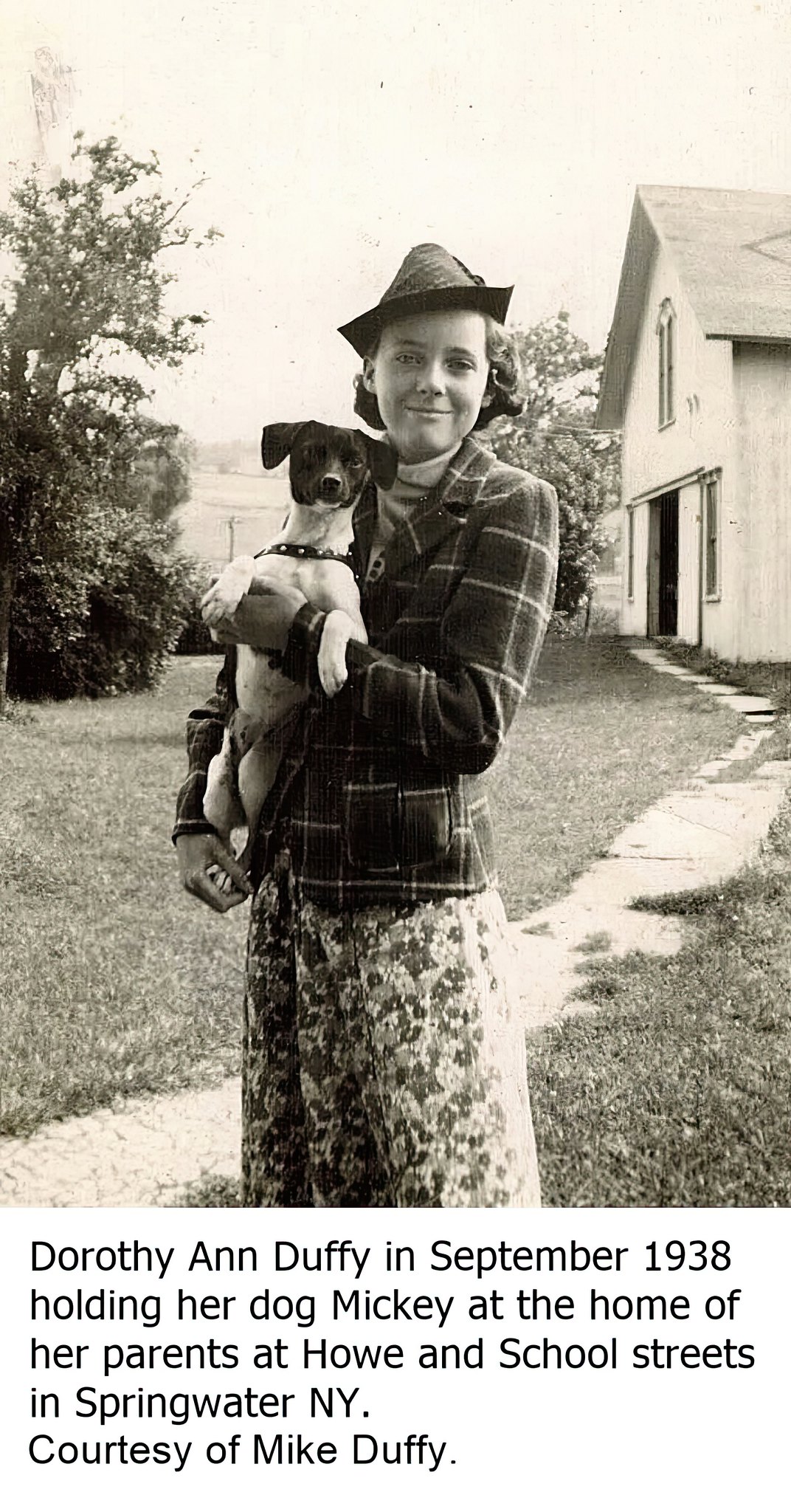In this older black-and-white photograph from September 1938, Dorothy Ann Duffy is seen holding her small dog, Mickey, at her parents' home located at Howe and School Streets in Springwater, New York. The picture, taken by Mike Duffy, captures Dorothy standing outdoors beside what appears to be a small house or cottage, possibly a barn, with a small stone pathway leading to it. The background features grass on either side and a few trees, suggesting it's either early spring or late fall given her attire. Dorothy, who appears to be in her mid to late teens or early 20s, is smiling happily. She wears a distinctive old-fashioned outfit, consisting of a plaid jacket with a collar over a floral print dress, and a small triangular-shaped hat with a little brim. Mickey, who resembles a terrier or Jack Russell with a black face and mostly white body, is cradled in both her hands, wearing a black collar adorned with white rivets. The photograph exudes warmth and nostalgia, beautifully preserving this moment from the past.